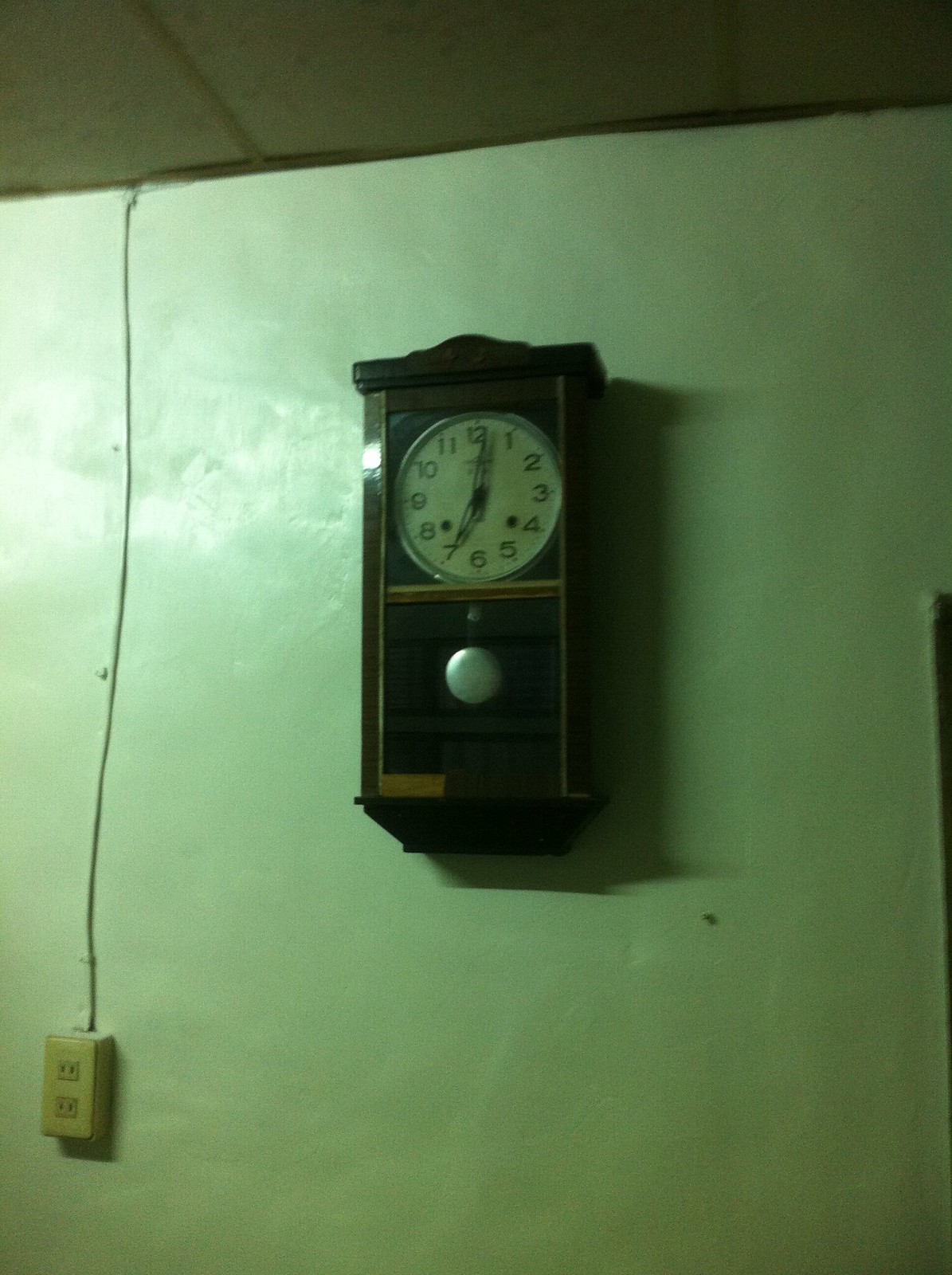This portrait-style photograph captures a wall-mounted, old-fashioned clock encased in a rectangular wooden box with tan accents and a front glass panel. The clock face, framed in silver, features a white background with black numbers and openwork black hands, indicating the time as 7 o'clock. A silver pendulum is visible in the lower compartment of the encasement. The clock is set against a plain white wall. To the left, there is an electrical outlet with an ivory faceplate, from which a wire extends vertically up the wall, adding a functional yet unobtrusive detail to the setting. The overall lighting in the room casts a slightly greenish-white tint, suggesting a low-quality image taken with a camera.